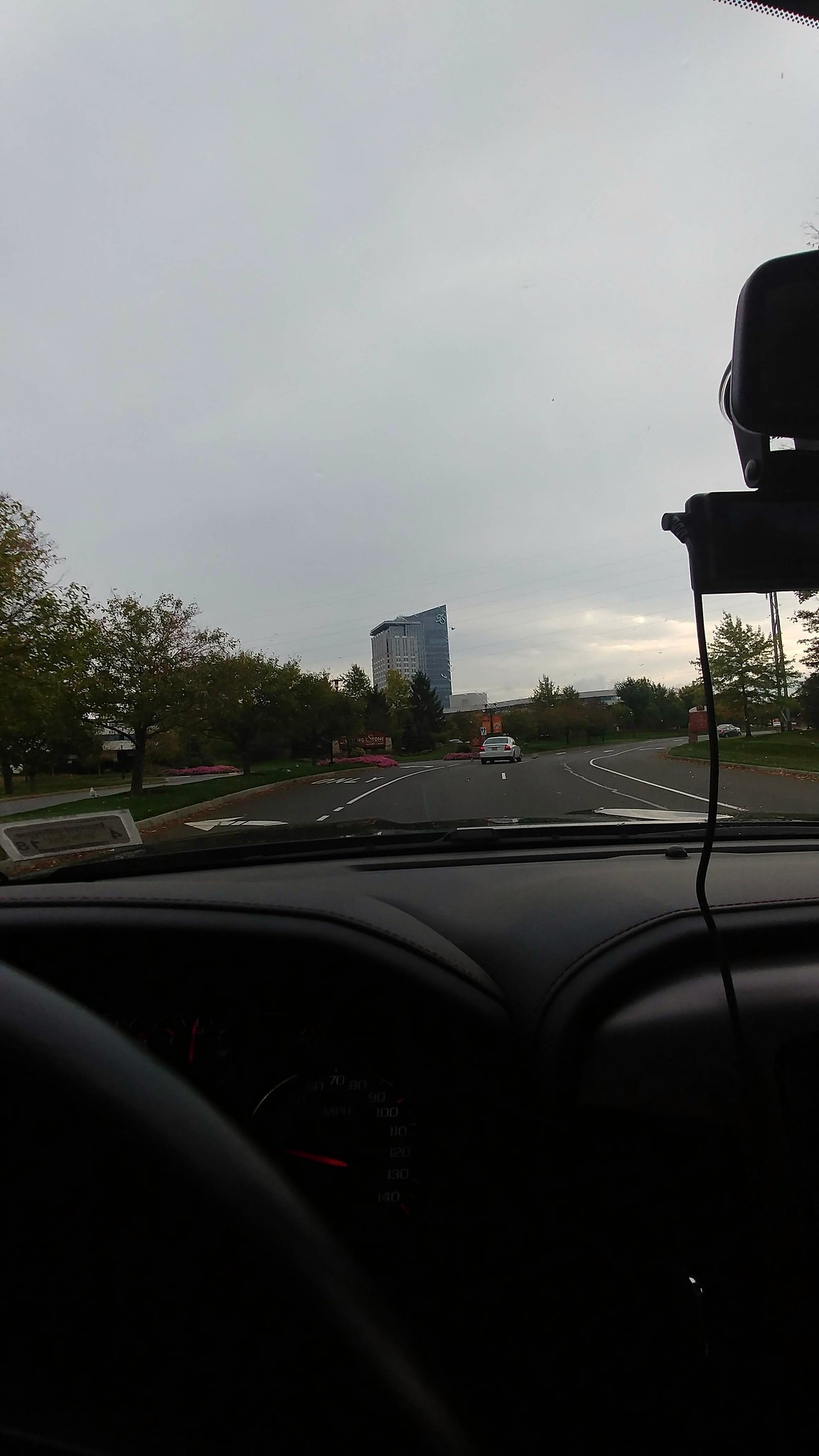This image is a photograph taken from the perspective of someone driving a car on a city street. The bottom portion of the image shows the dark, shaded interior of the car, including a black steering wheel and dashboard. In the upper right-hand corner, a device—possibly a cell phone or dash camera—hangs from the windshield with cords attached. Through the windshield, you see a gloomy gray sky stretching over the scene, indicating an overcast day.

Ahead, a large rectangular building with an angled top dominates the skyline, suggesting it might be a combination of two structures—a gray one in front and a bluish one behind. In the far distance to the right, you can spot a red truck, likely on a highway that runs parallel to the road you are on. 

Closer to the foreground, the photograph reveals a two-lane road curving slightly to the right, with a white car up ahead and another vehicle crossing the road. To the left, a line of trees, grass, and a pathway follows the road's curve, emphasizing the greenery. There are additional street details, such as a left turn lane, a median strip dividing the highway, and signs that might include a telephone pole. The overall atmosphere is somewhat dim, reflecting the late-in-the-day lighting.